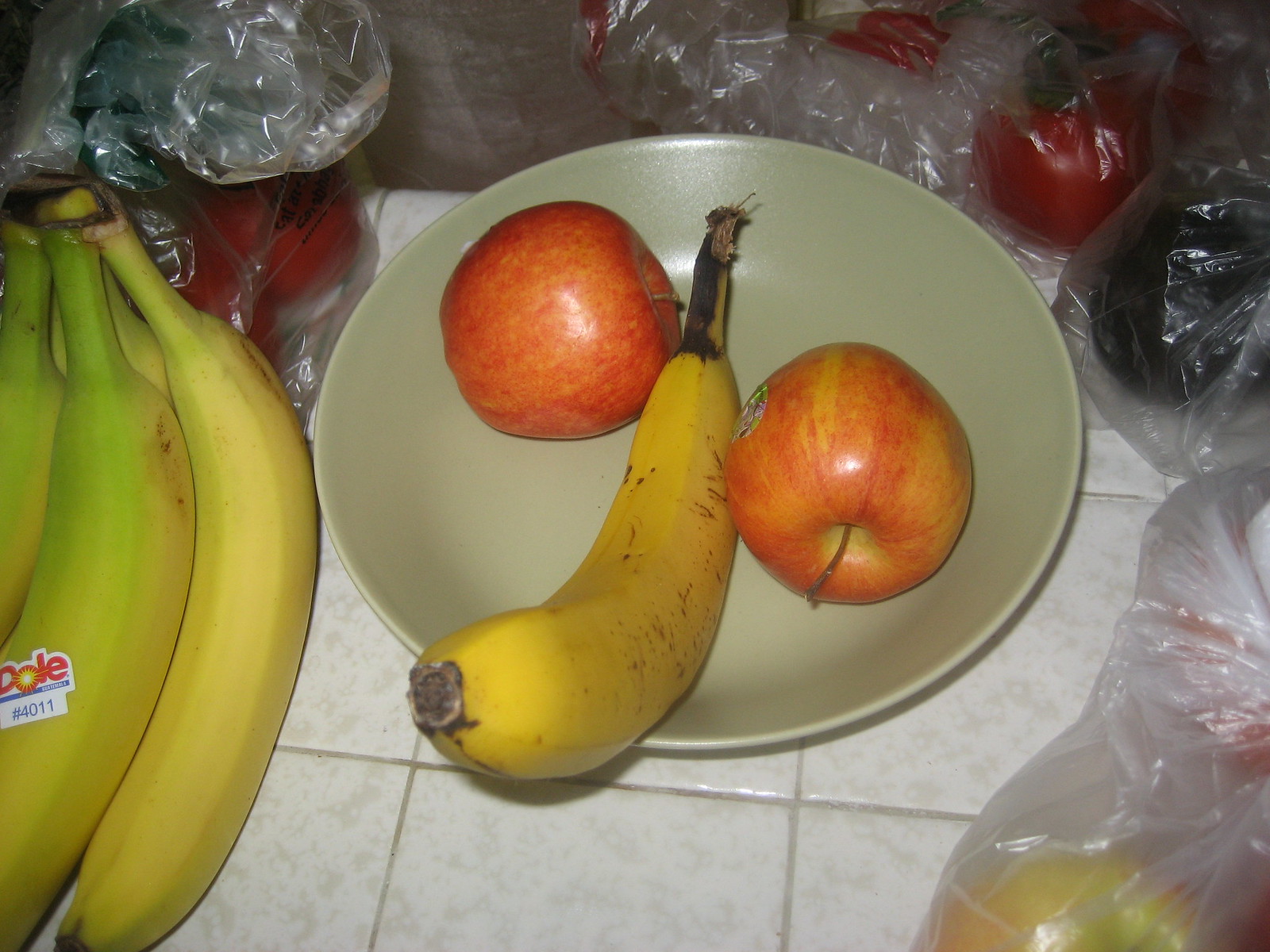In the center of the image, a shallow, greenish eggshell-colored ceramic bowl holds a single banana laid on its back, curving up and out of the bowl's edge. Flanking the banana are two red apples, one on each side. This bowl is placed on white tiles with gray grout lines. To the left, a bunch of bananas rests on the tile floor, with a plastic bag containing red fruit in the background. On the right side of the photo, the top right corner features more red produce in a plastic bag, with darker produce—possibly avocados or plums—just below it in another bag. The bottom right corner contains what appears to be more apples in a plastic bag. The composition is striking, with the central bowl of fruit framed by additional produce, creating a vivid display of color and texture.